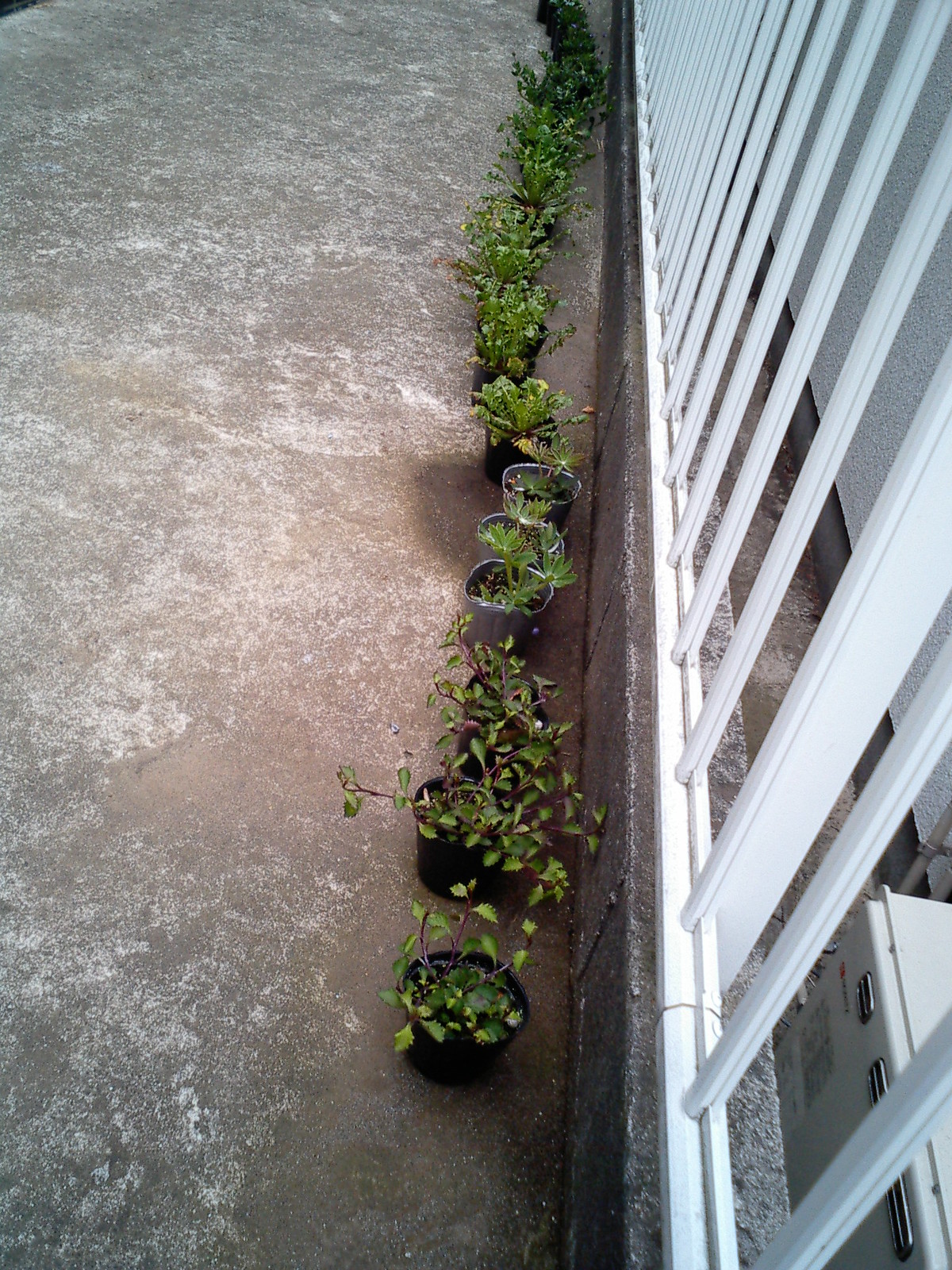This color photograph captures a line of small, predominantly green plants in black and grey pots, situated on a light grey cement floor adorned with white speckles. The plants, featuring brownish stems, stretch upward and outward, with some appearing slightly wider than others. They are positioned along a greyish half-wall, above which stands a white metal fence with vertical bars. The line of plants, consisting of about a dozen seedlings and young ivies and ferns, begins towards the forefront middle of the image and extends to the top middle, creating a rhythmic visual along the fence. In the background, behind the railing, a large heating element with pipes is partially visible, adding an industrial touch to this residential or commercial setting.